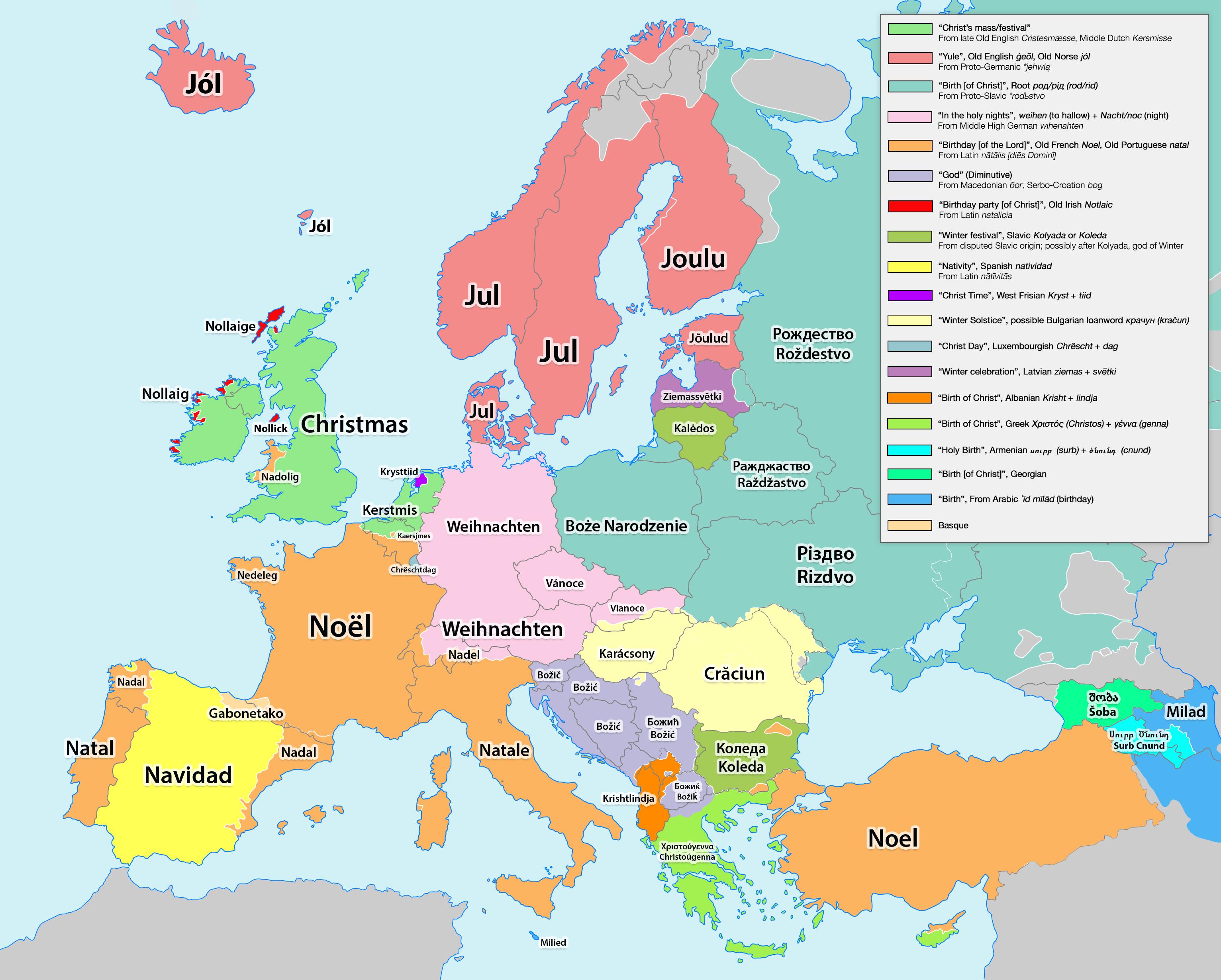The image features a detailed map depicting much of the world, highlighted by a legend on the side. The map is vividly color-coded to represent the different words used to denote Christmas across various regions. Each color corresponds to a specific term for Christmas. 

- **Pink** indicates regions where Christmas is referred to as Jol, Jul, Joulu, Julu, or other variations of Jul.
- **Green** signifies areas where the term "Merry Christmas" is used.
- **Yellow** highlights regions, primarily in the west-southern parts, where the term "Navidad" is used.
- **Brown** is used to show areas that refer to Christmas as Natal, Noel, or Natali.
- **Purplish color** represents regions where the term "Wynachton" is prevalent.
- **Beige color** indicates places where Christmas is called Crecyon.
- **Bluish color** is used for regions where the term "Rosedestvo" is common.
- Additionally, another term for Christmas, "Milad," is also mapped out.

The map offers a comprehensive and colorful overview of the diverse names for Christmas celebrated around the world, accompanied by corresponding regional color codes for easy reference.